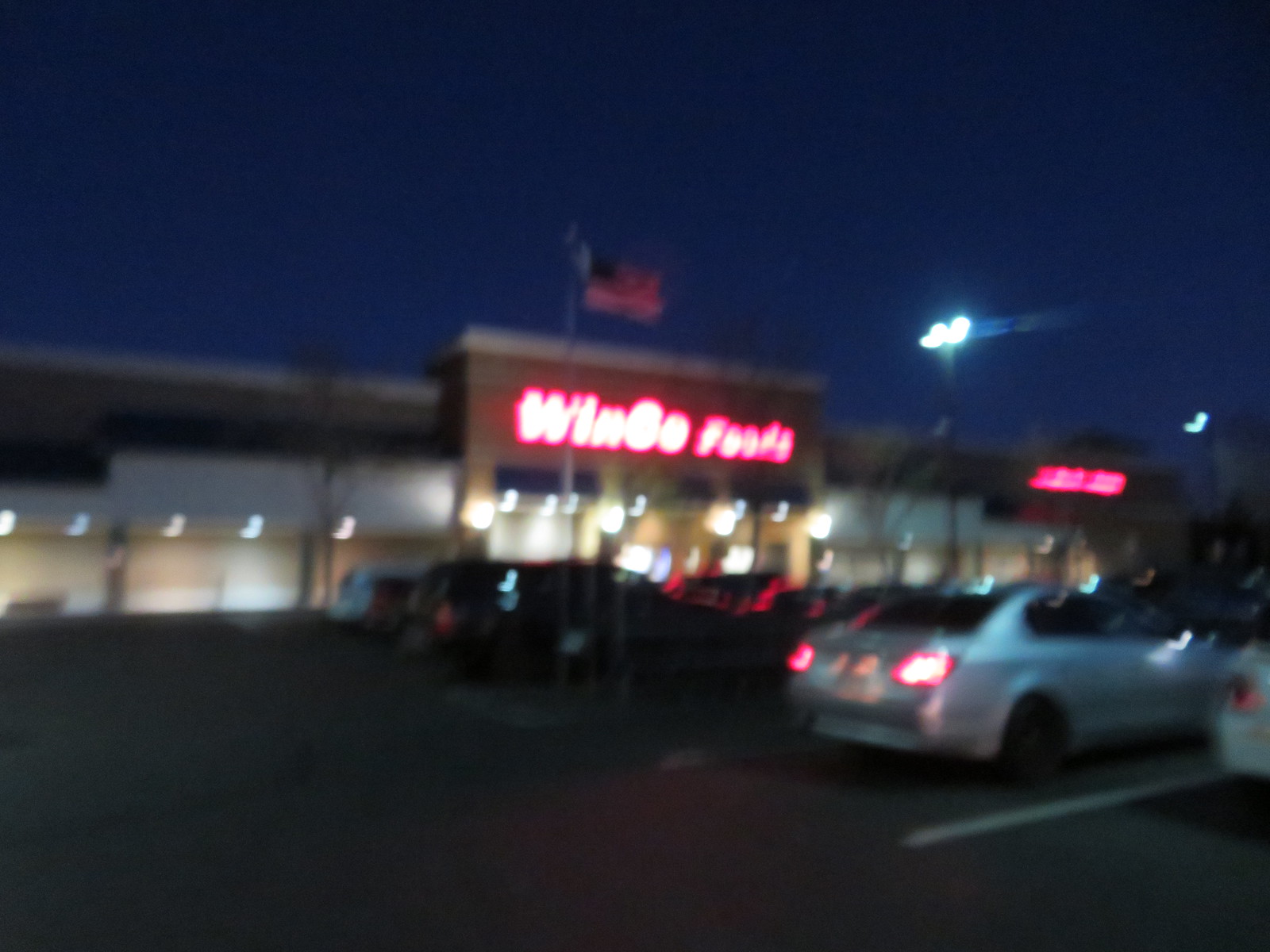This color photograph captures a blurry nighttime scene of a car park. At the bottom of the image, several white lines marking parking spaces are visible on the right side. A line of cars is seen parked, with a grey car closest to the camera, its red taillights glowing. In the background, a large building is prominently featured, displaying an American flag atop it. There is a red sign on the building with a partially legible "W" at the front, possibly spelling out 'Windy Park.' Multiple lights adorn the building, suggesting it is well-illuminated. A streetlight is positioned towards the right, appearing slightly blurred. On the far right, a crescent moon is faintly visible against the very dark blue night sky.